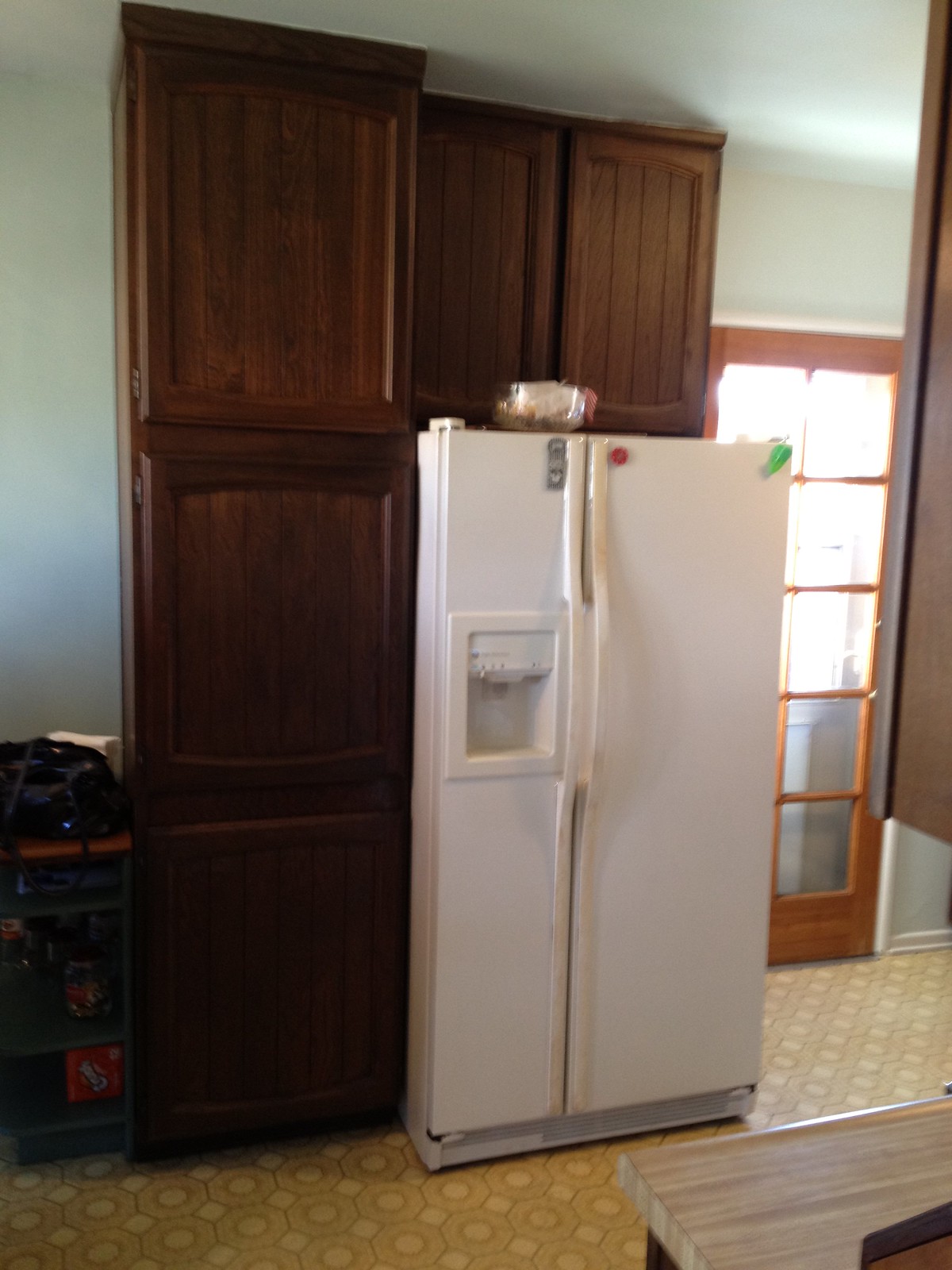This color snapshot captures a dated, somewhat drab kitchen space that's likely in a house or apartment. Prominent in the center of the image is a large, white two-door refrigerator with an ice and water dispenser inset on the narrower left side door. The top of the refrigerator is cluttered with food items wrapped in cellophane, and there are a few magnets adorning its upper section. Surrounding and surmounting the fridge, there's a series of dark brown, grainy cabinets: three vertically aligned on the left, and two horizontal cabinets at the top, reaching up to the ceiling. 

To the refrigerator's right, there's a wooden door with sunlight filtering through its ten inlaid glass panels. The kitchen floor is covered in an octagonal patterned linoleum that's beige and light brown, showing signs of wear. In the lower right corner of the image, a wooden table corner and a Formica kitchen countertop with an overhead brown cabinet are partially visible. The bottom of the refrigerator features a grate, emphasizing its older style, and reinforcing the room's overall lived-in feel.